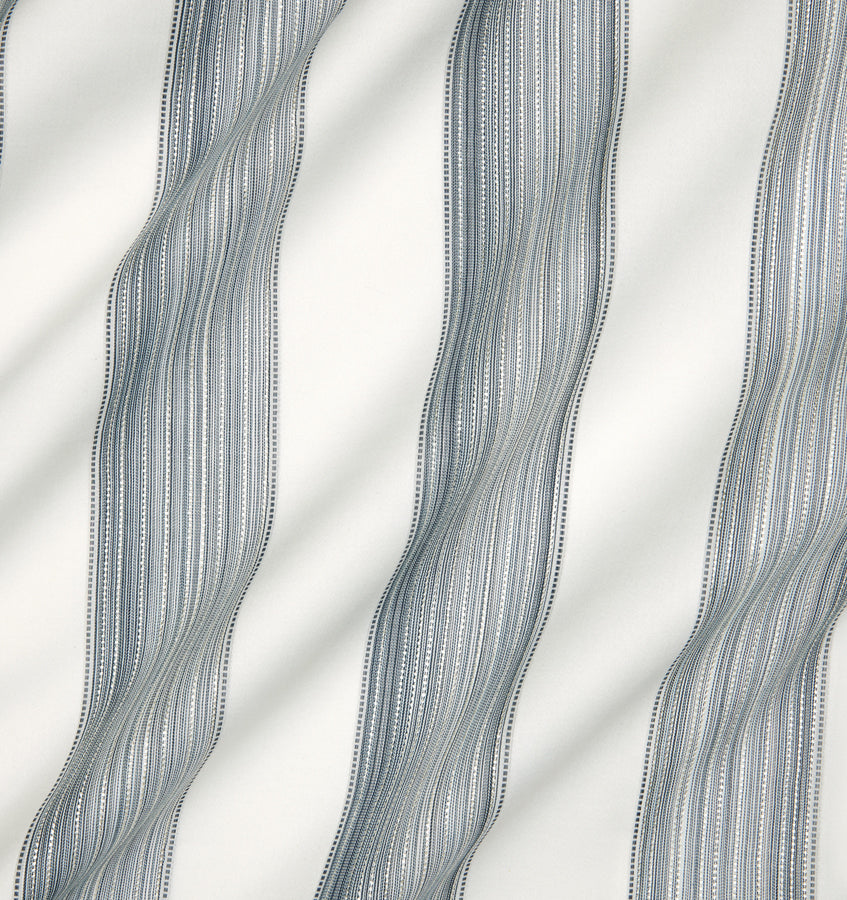The image depicts a piece of fabric, likely satin, with intricate and elegant detailing. The material is predominantly off-white, resembling the luxurious feel suitable for a wedding or prom dress. There are three prominent pale gray stripes running vertically down the fabric, giving it a structured and refined appearance. These stripes vary in opacity, with some being solid gray while others are more translucent, allowing the white background to show through. Bordering these stripes are tiny, nearly black dots, which create a delicate ribbon-like effect. The design is uniform throughout the fabric, with the stripes and dot patterns repeating consistently. This intricate detailing and refined material suggest it could also be used for high-end bed linens, highlighting its versatile elegance.